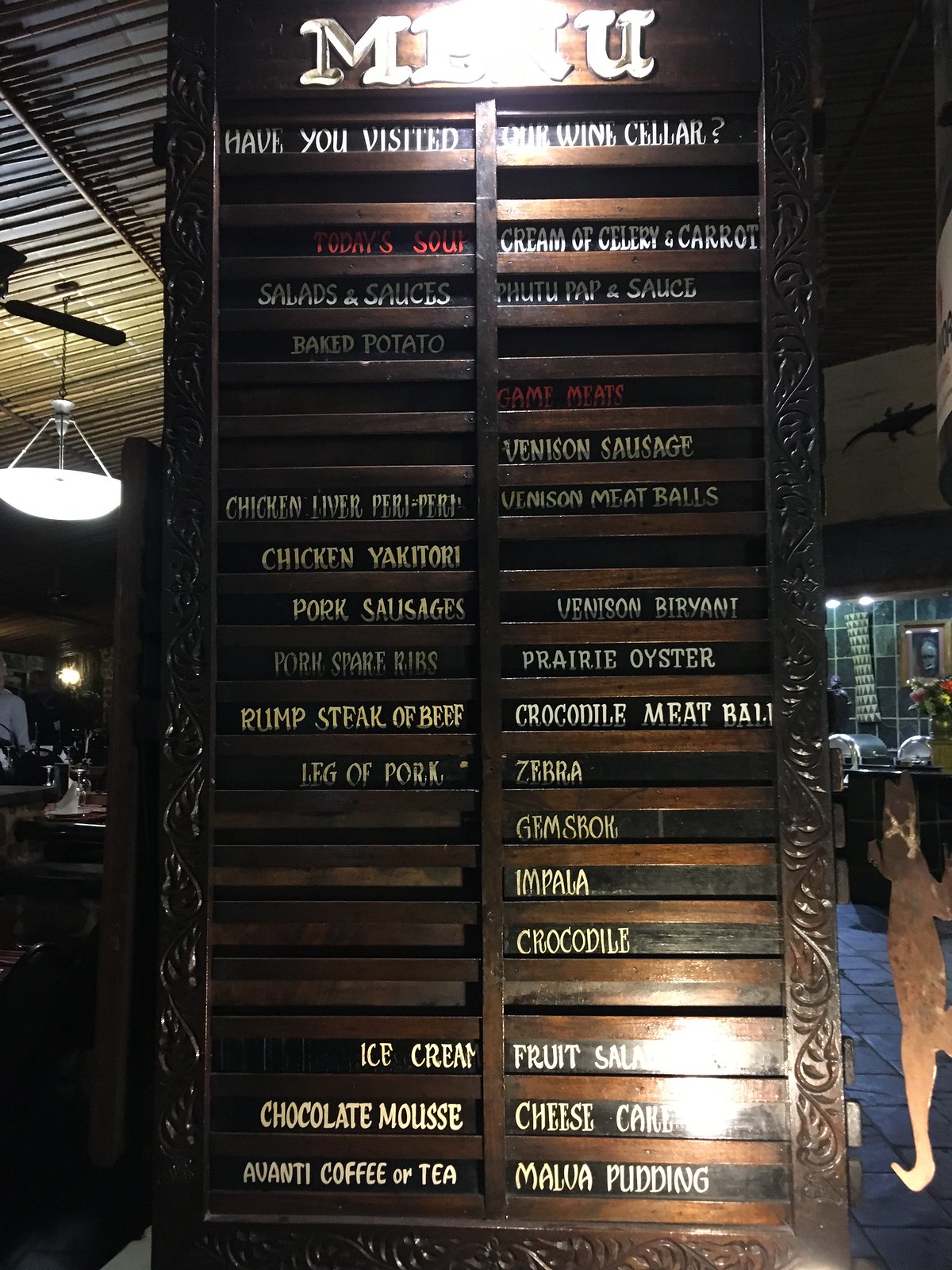Inside a rustic restaurant, the stone floor exudes a warm, earthy feel. In the background, a bar area is partially visible, adding to the cozy ambiance. Dominating the scene is a large, wooden board with intricate carvings and detailed information. At the top, white carved letters ask, "Have you visited our wine cellar?" Below, in striking red letters, the daily special is announced: "Today's soup, cream of celery and carrot." The board continues to outline an extensive and diverse menu including salads, sauces, baked potatoes, and an array of exotic game meats such as venison sausage, venison meatballs, chicken liver, chicken yakitori, pork sausages, pork spare ribs, beef rump steak, leg of pork, prairie oysters, crocodile meatballs, zebra, and impala. For dessert, options like ice cream, chocolate mousse, Malua pudding, cheesecake, and fruit salad tempt the patrons, topped off with a choice of Avanti coffee or tea.